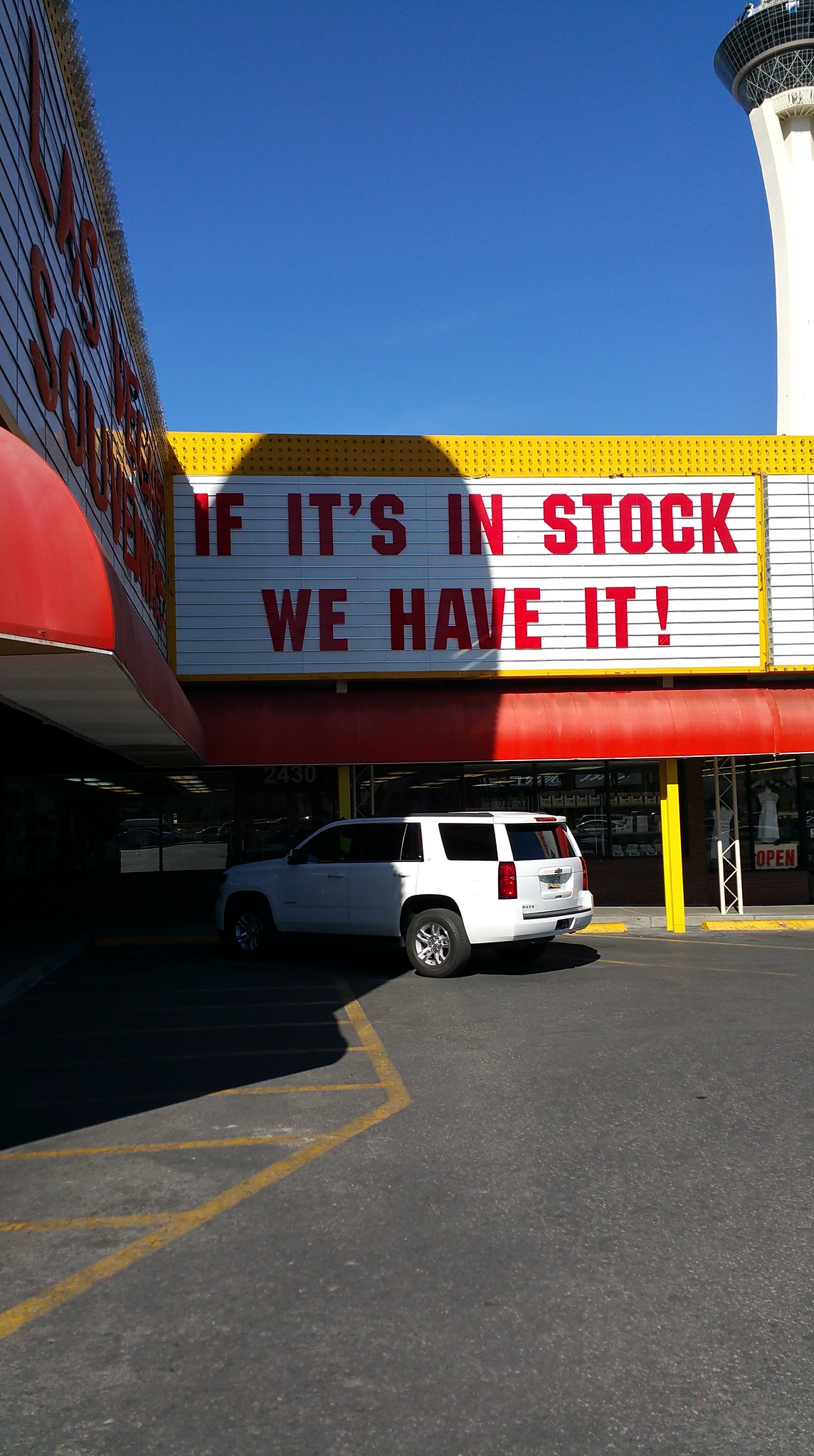This photograph showcases the exterior of a store, presumably located in Las Vegas, possibly named "Las Vegas Super Store" or "Super Center," inferred from the partially obscured red capitalized writing against a white background on the left side of the image. The text is angled awkwardly, making it difficult to decipher completely. 

Prominently displayed on the front side of the building is another sign, also featuring red capitalized writing on a white background, bordered in yellow. The sign reads, "IF IT'S IN STOCK WE HAVE IT!" The yellow border appears to be adorned with lights, suggesting it may be illuminated during the night.

Parked beneath this sign is a white SUV, which is turned off. To the right of the building, a small "OPEN" sign is visible, following the same white and red color scheme. Above this sign, there is a plastic mannequin dressed in a short, white summer dress.

The photograph was taken on a bright, sunny day with clear blue skies and no clouds. In the background, on the right side of the image, there is a distinctive white tower with a curved design, featuring a black band encircling it.